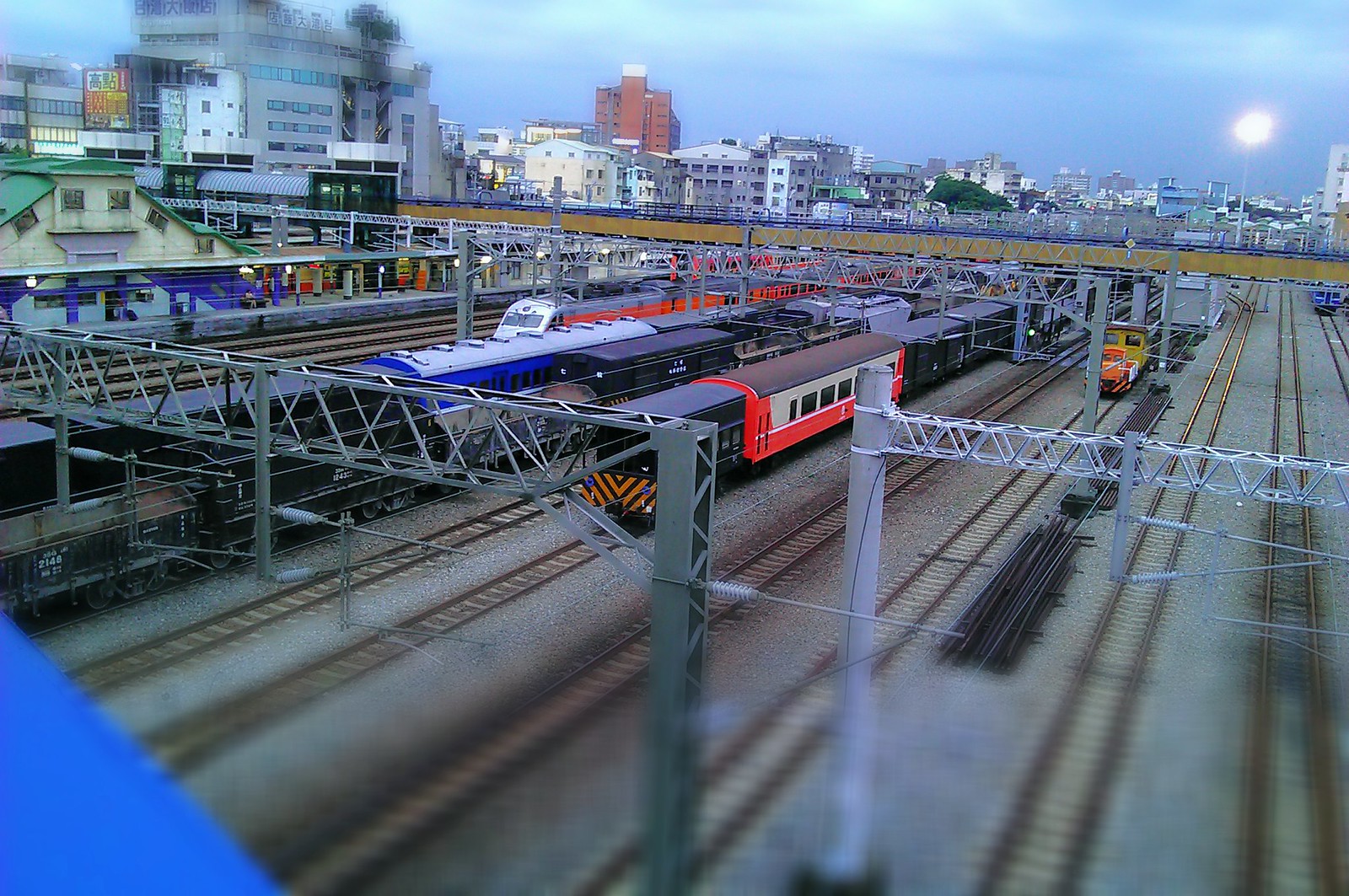The image depicts a large railroad yard at twilight, with a significant blue hue that may indicate a blue filter or twilight lighting. There are six parallel sets of train tracks, each occupied by trains of varying lengths, with three of the trains on the leftmost tracks extending partly out of the frame. The locomotives of two of these trains are visible. In the foreground, the tracks are blurry and out of focus, while a bright blue triangle, possibly part of a sleeve or building, occupies the lower left corner.

The yard features overhead steel truss frames and multiple lights, underscoring its industrial nature. On the left, a passenger platform is visible, with a covered waiting area. Additionally, a pedestrian bridge spans across the yard, possibly connecting to another cropped-out platform on the opposite side. In the background, a medium-sized urban cityscape is visible against a sky that, despite its dark and twilight appearance, is illuminated by a large white globe light or possibly the sun obscured by clouds, located in the upper right corner of the frame. Overall, the image captures the bustling and structured environment of a city train station transitioning between day and night.